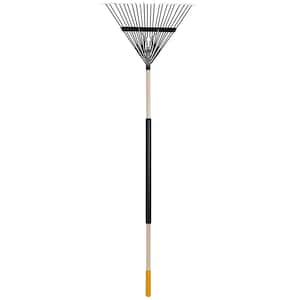The image features a simplistic depiction of a leaf rake standing upright on a plain white background. The rake is positioned upside down, with its handle touching the ground and the metal tines pointing upwards in a fan shape, creating a V or Y appearance. The handle of the rake has several distinct color sections: the tip is yellow, followed by white, then a long black section, another white segment, and finally a small black segment before transitioning into the metal tines. The tines are held together by a horizontal black bar for added stability. The photograph, or possibly an illustration taken from a distance, emphasizes the rake as the sole focus of the image, with no other elements or background details to distract from it.